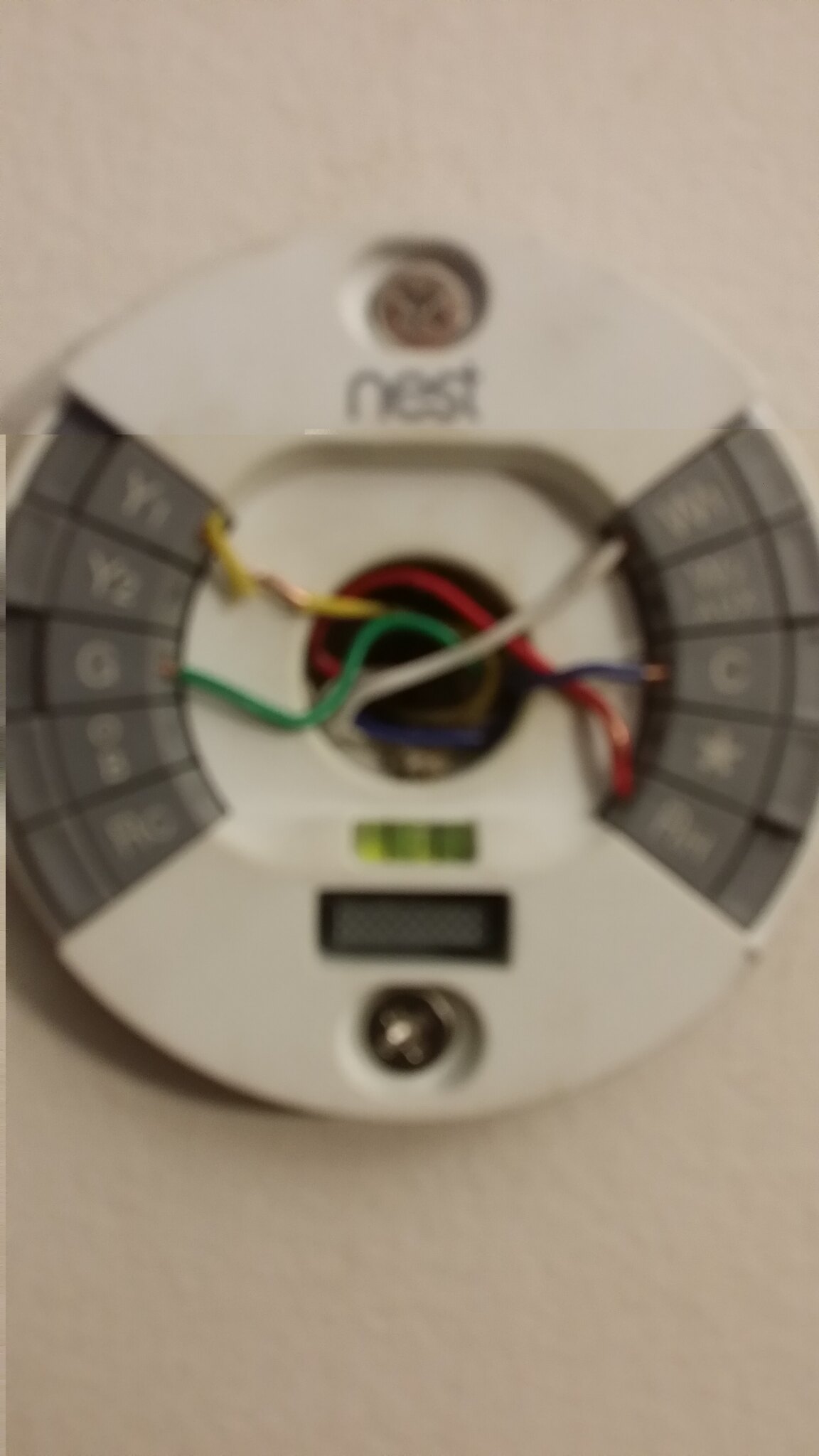The photograph captures a close-up view of a device mounted on a white wall. The image is notably blurry, but several details are discernible. At the center of the circular device, there is a cutout section filled with a bundle of wires in various colors: white, red, green, yellow, and what appears to be either blue or purple, making a total of five wires. 

On the right-hand side of the device's rim, there are various buttons or wire connectors, each labeled with different symbols and letters. At the top, there's a button labeled with a "W," followed by an unreadable label beneath it. Continuing down, the buttons are labeled "C" and then another featuring a star symbol. The next button's label is illegible.

On the left-hand side of the device, buttons are labeled "Y1," "Y2," "Q," and another illegible symbol underneath them. At the very top of the device is a rusty screw, and just below that, the word "Nest" is printed. Below the central cutout section harboring the wires, there's a neon green square, underneath which lies a black-rimmed square with a gray interior. Another area below this square holds a silver screw, which shows less rust compared to the screw at the top of the device.